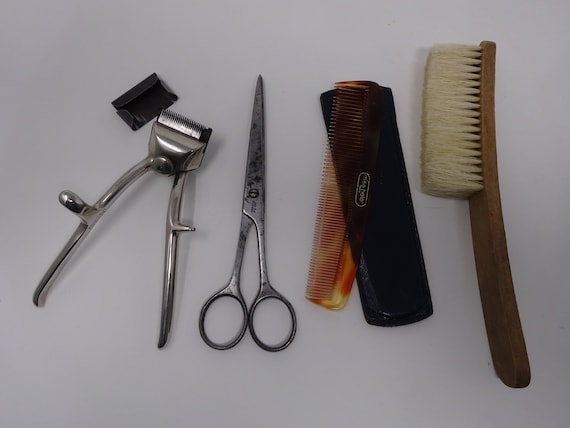This image showcases a curated set of antique barber tools laid out on a whitish gray surface, likely intended for a vintage sale. Starting from the right, there is a wooden-handled brush with coarse, long, yellowish-white bristles. The brush’s handle is made of dark brown wood and has a gently rounded back. Moving left, we find two stacked combs: the top one being a dark brown and the bottom featuring lighter brown and yellowish swirls. To the left of the combs lies a pair of well-worn, silver hair-cutting scissors, showing signs of rust. Further left, in the center of the image, sits an antique silver buzz cutter with a small black sheath to cover the blades when not in use. This clipper features two handles with distinctive finger nubs for grip, emphasizing its old-fashioned design. The careful arrangement and vintage condition of these tools evoke a bygone era of traditional barbershops.